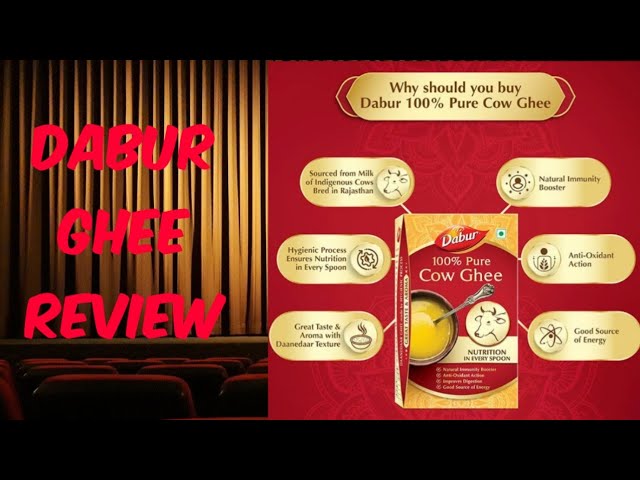The image appears to be a paused screenshot from a review video or an advertisement for Dabur 100% Pure Cow Ghee. The setting to the left features a theater-like atmosphere with red, perhaps velvet, seats, and a stage adorned with vertical golden-yellow curtains. Dominating the right side of the image is a vibrant red and black graphic area, which contains key promotional information for Dabur Ghee.

In large, all-caps red letters, the graphic reads "DABUR GHEE REVIEW," followed by a headline stating, "Why You Should Buy Dabur 100% Pure Cow Ghee." Below this, the product is prominently displayed in its predominantly orange and red packaging, accompanied by an image of the bright yellow clarified butter and a picture of a cow highlighting "nutrition in every spoon."

Surrounding the product are gold-rounded text shapes elaborating on its qualities: sourced from the milk of indigenous cows bred in Rajasthan, ensuring nutrition through hygienic processes, great taste and aroma with Dhaneda texture, natural immunity-boosting properties, antioxidant action, and being a good source of energy. Some smaller, illegible text is present, likely providing additional details or disclaimers.